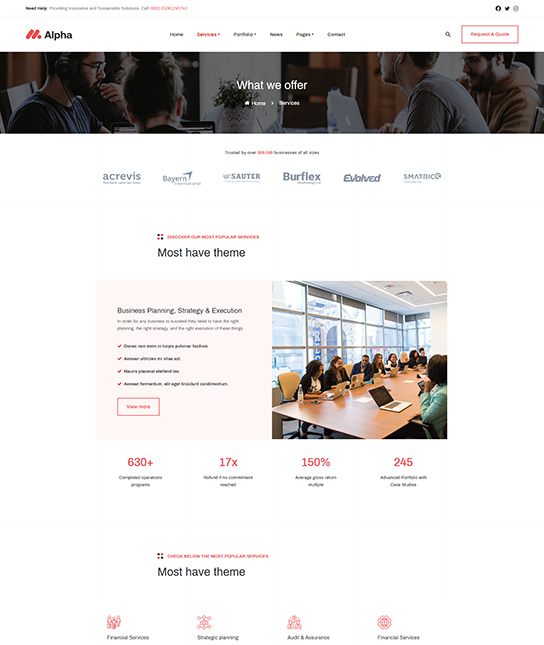The main image showcases the homepage of a website. In the top left corner, the word "Alpha" is prominently displayed. To its right, there is a stylized red symbol. The navigation menu includes options labeled "Home," "Services," "Portfolio," and "News," among others, though the exact content beyond "News" is unclear. The "Services" tab is highlighted in red, indicating it is currently selected. 

On the far right of the navigation bar, there is a magnifying glass icon suggesting a search function, and a "Request a Quote" button. 

Below this navigation bar, headings such as "Acrobis," "Bears," "Salter," "Burflex," "Involved," and "Symmetric" can be seen, likely representing sections of the website or key service areas. A prominent tagline in red text reads "Business Planning, Strategy, and Execution."

To the right, there is an image of people sitting around a meeting table with large glass windows in the background, giving the scene a bright and open atmosphere. Additionally, numerical statistics such as "630+" (perhaps projects completed), "17x" (possibly growth factor), "150%" (maybe efficiency gain), and "245" (likely client count) are highlighted, though their precise meanings are not specified.

Below these elements, more sections are delineated with red text headings and various other subheadings and content. The page is rich in detail and features various thematic elements marked in red to capture attention.